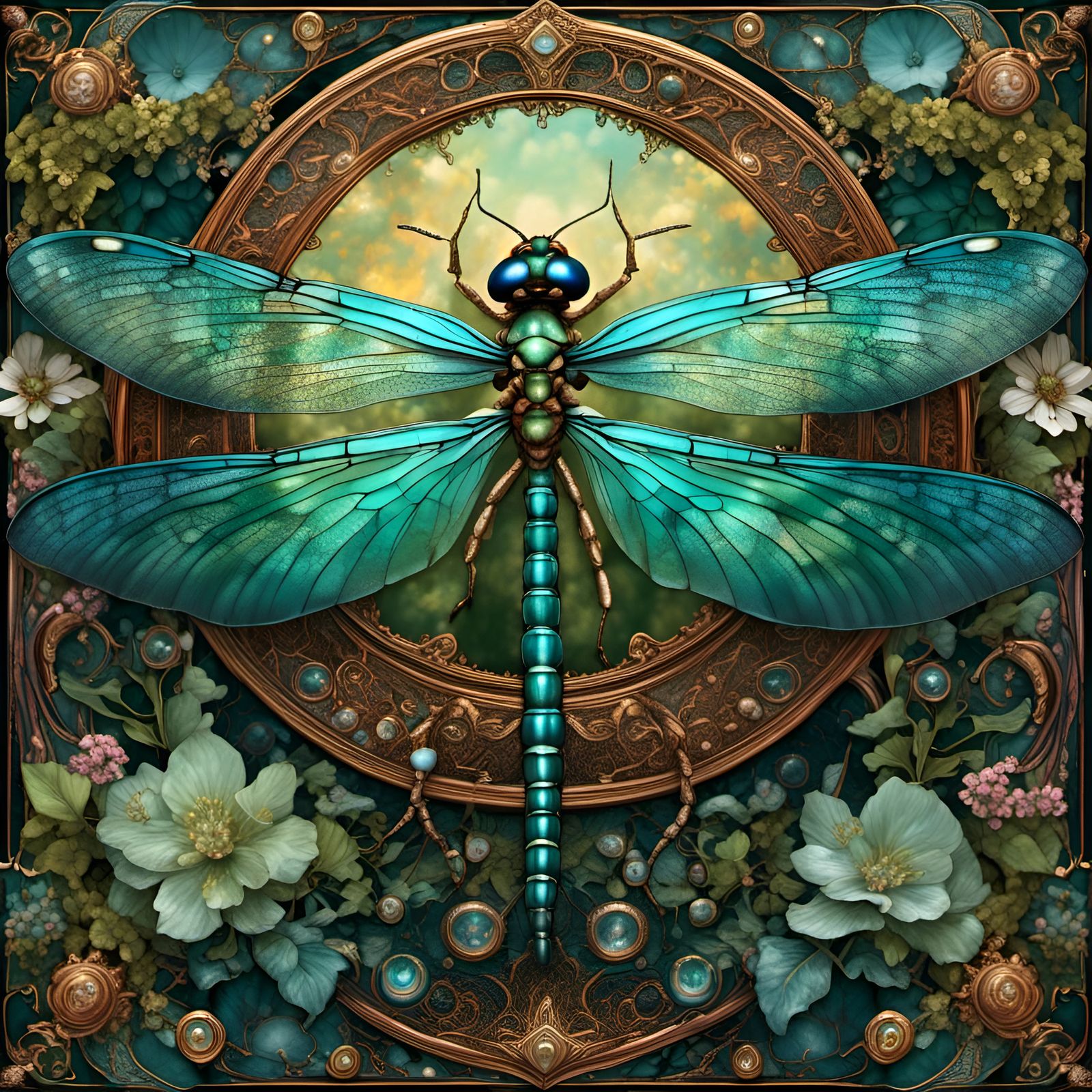This captivating image showcases an intricate artistic rendering, possibly a computer-generated image or painting, of a decorative dragonfly. The dragonfly dominates the composition, facing from the top side of the image to the bottom. It features a beautifully segmented green tail adorned with horizontal golden stripes and a body that blends earthy browns with green hues. The dragonfly's eyes are a vivid blue, and it has two delicate antennas.

The creature boasts two sets of azure wings; the upper wings are slightly translucent, while the lower wings appear more solid. The entire dragonfly rests on an ornate bronze ring with swirling, trellis-like metalwork and embedded turquoise jewels. This ring serves as the centerpiece of the image, surrounded by a lush green background and vibrant flowers in shades of white, teal, and bronze, with touches of pink. The floral embellishments appear almost three-dimensional, with some bronze metal swishes and beading adding to the decorative complexity. The overall color palette is a harmonious mix of blues, greens, and bronzes, enhanced by strategic lighting that highlights specific details, creating a visually stunning, richly detailed work of art.